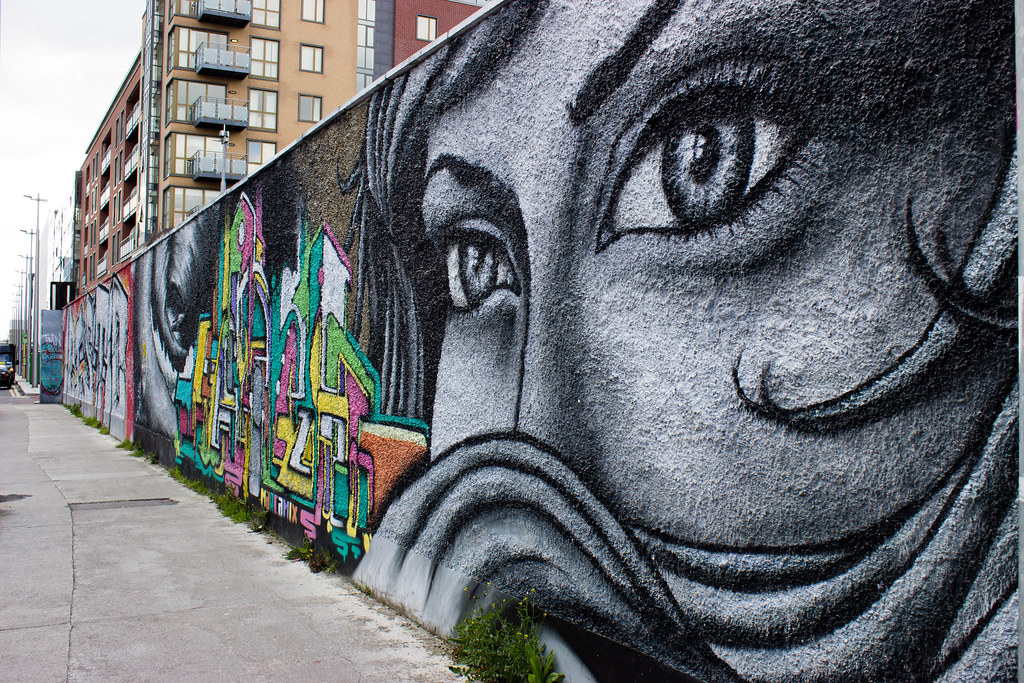The photograph captures a vibrant outdoor scene, focusing on a long concrete wall adjacent to a sidewalk on the left. The wall, which tapers as it extends from right to left, serves as a canvas for a series of murals. Dominating the right side is a striking black and white close-up of a woman's face, her long hair swirling and partially obscuring her mouth, creating a sense of mystery. Adjacent to this portrait is a vivid burst of graffiti, featuring colorful, intertwined letters rendered in greens, yellows, and pinks. Further along, another monochromatic image, possibly of a man, is painted in black and white. This is followed by more graffiti in red and white hues, though the exact words are indiscernible. Above the wall, the background reveals tall apartment buildings in shades of red, tan, and gold, set against an overcast sky. In the lower part of the image, overgrown plants and weeds line the base of the wall, adding a touch of untamed nature to the urban setting. On the far left, a dark-colored vehicle is parked, completing the vivid, eclectic urban tableau.